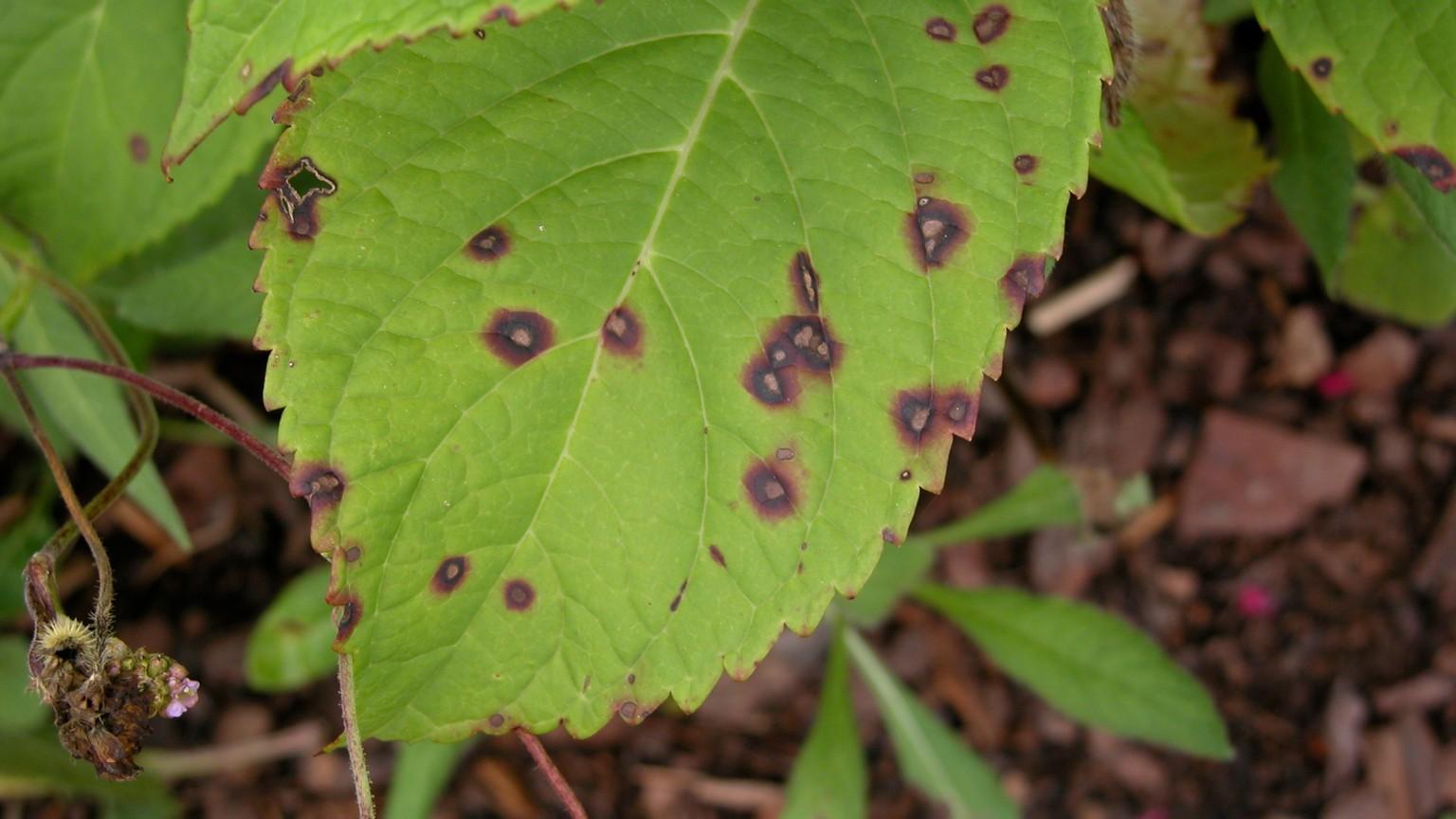This image is a detailed, close-up photograph taken outdoors during the daytime, depicting a single green leaf with distinct signs of disease or damage. The leaf, with light green veins and serrated edges, occupies the central two-thirds of the picture from the top to the bottom. It is marked by approximately 20 dark red dots, each with light tan centers that transition into very dark, nearly black borders, and then fade into rust-colored edges. Surrounding this main leaf, there are partial views of other similarly affected leaves. The background features a slightly blurred forest floor covered with brown mulch, dead leaves, and hints of muddy, humid conditions. Additionally, a rotten flower is visible on the left side. The overall color palette includes bright and dark greens for the leaves, various shades of brown for the ground, and the distinctive coloring of the damaged spots.